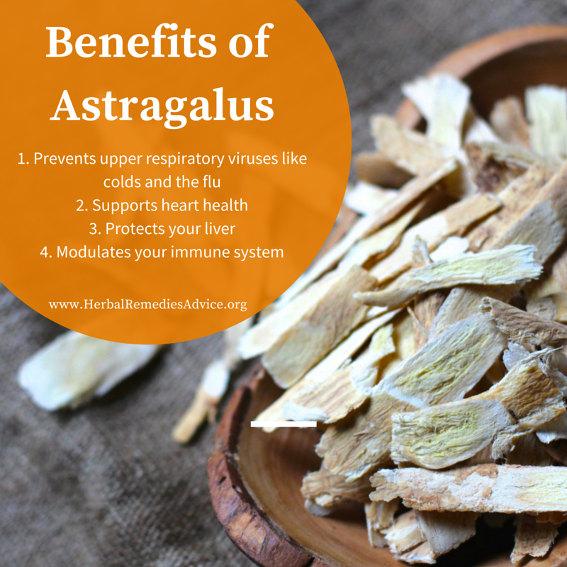The image features a rustic, round wooden bowl filled with freshly chopped or shaved bright-colored astragalus root, complete with tree bark fragments, placed atop a gray or natural-colored burlap sack. Positioned predominantly on the right side of the image, the bowl contrasts with the promotional text on the left. The text is enclosed within an orange circular thought bubble and is written in white, detailing the benefits of astragalus: "Prevents upper respiratory viruses like colds and the flu, supports heart health, protects your liver, and modulates your immune system." The website www.herbalremediesadvice.org is also included. The overall composition suggests this is a page from a brochure or a promotional poster, emphasizing the herbal remedies of astragalus.